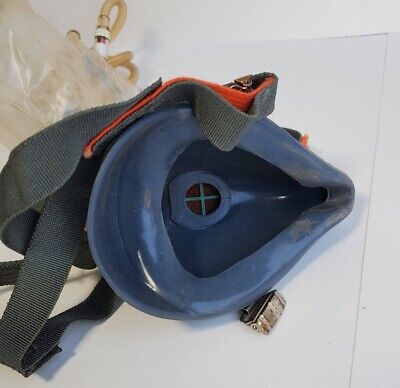The image depicts a well-worn, navy blue silicone dusk mask, possibly used for woodworking or other dusty activities. The mask has black and red Velcro straps, which appear to be secured to a black case. The mouthpiece of the dusk mask shows signs of use with visible dust particles. It is lying on a white tabletop. In the background, there are various elements related to plumbing, including a clear plastic bag and various types of rubber and plastic tubing. Additionally, there's a silver component attached to the black case, and some elements appear to be set against a background that could resemble a plastic shower curtain. This combination of tools and equipment suggests a detailed, albeit cluttered, workspace.